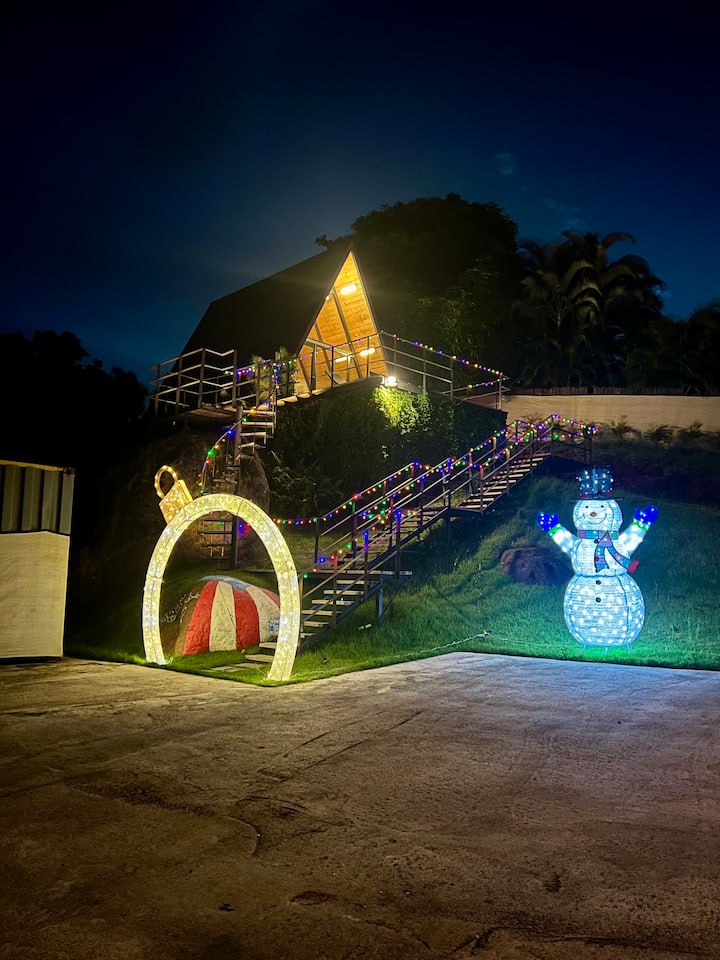This photograph captures a festive scene, most likely set at dusk in either a residential property or a public park adorned with Christmas decorations. Dominating the background is a striking, A-frame, triangular wooden structure atop a hill, bathed in warm lighting. This structure, standing on a platform with railings, is approached via a series of steep stairs illuminated with twinkle lights in hues of blue, purple, green, red, and yellow.

At the base of the stairs, a lit-up archway resembling a golden Christmas ornament creates a welcoming entrance. Adjacent to the second set of stairs, there stands a charming snowman made of lights, glowing white with blue gloves and a top hat, adding a whimsical touch to the scene.

In the foreground, the viewer's perspective is anchored by a grey pavement or possibly a driveway, void of cars, and a patch of grassy area where the snowman is placed. The sky above is a deep blue, signaling the onset of nightfall and allowing the vibrant Christmas lights to shine brightly, amplifying the festive atmosphere.